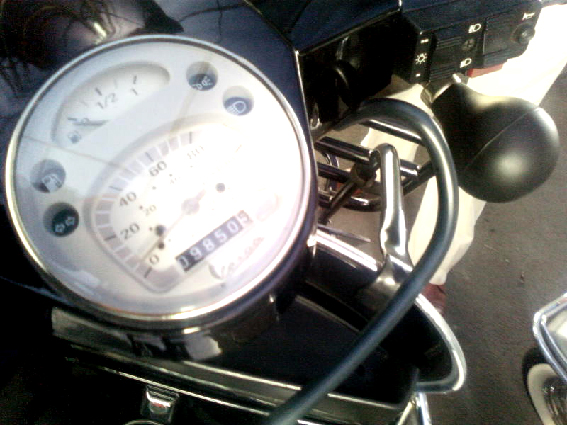This photograph captures the instrument panel of a motorcycle from the rider's perspective, looking downward at the controls. Dominating the left side of the panel is a large white dial, marked from 0 to 1, serving as the fuel gauge. At the top of this dial, a classic gas pump icon further indicates the fuel level. Flanking this, smaller icons depict left and right turn signals with arrows, and lights facing outward on both sides. A larger light symbol indicates the high beams, all set against a black background with stark white icons for clarity.

Central to the panel is an expansive dial, calibrated from 0 to 100, displaying the motorcycle's speed in large, easy-to-read numerals. Nestled within the speedometer is the mileage counter, currently displaying 9850 miles.

The right side of the instrument cluster features a black control panel housing various instruments, including a prominent horn button designed to be activated by a squeeze, along with other elements crafted from chrome and polished black metal. The entire setup rests on a concrete surface or within a parking lot, grounding the scene in a practical, everyday context.